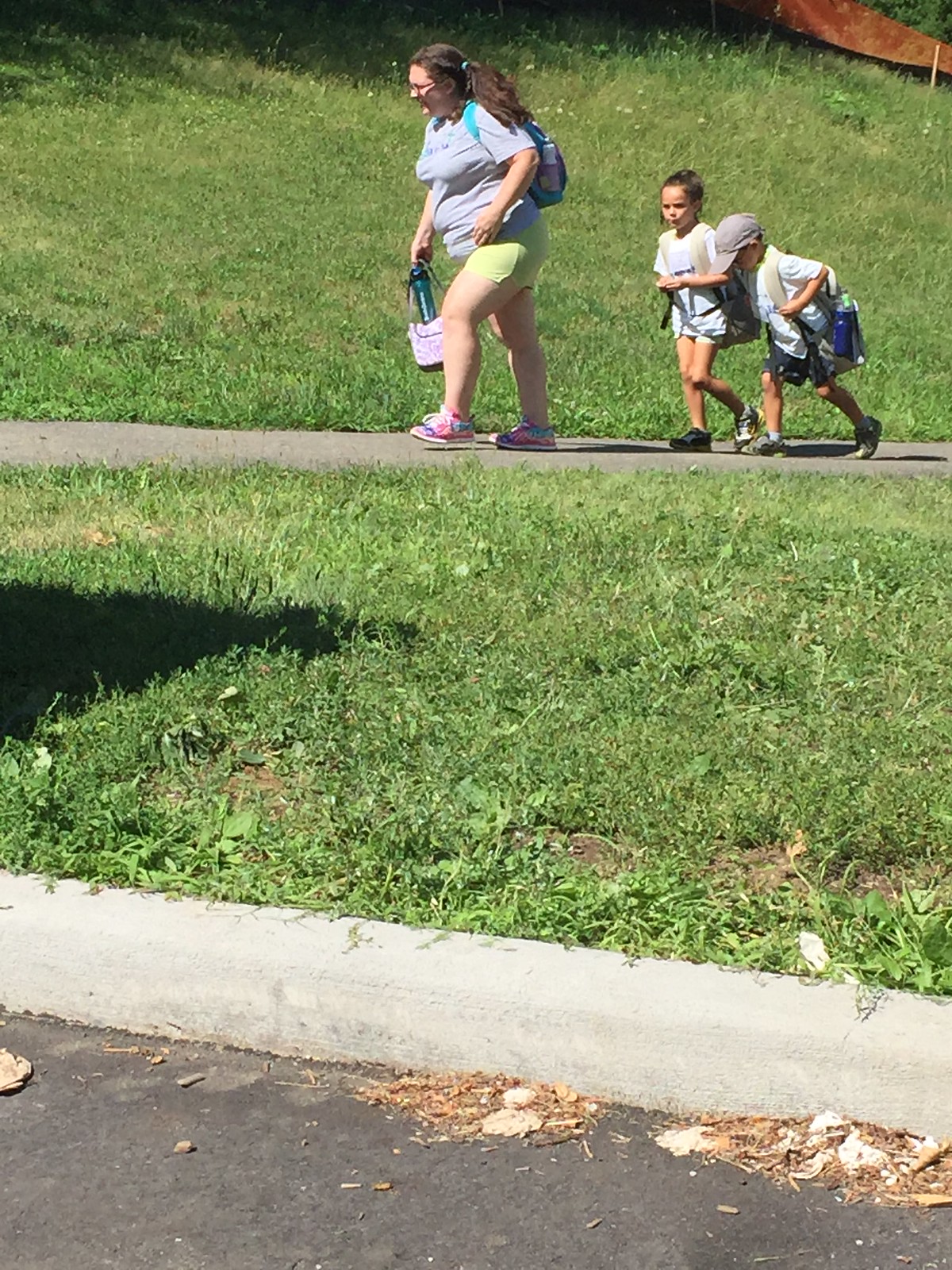The photograph captures a family as they walk uphill along a gray concrete path that cuts through a grassy park area. In the foreground, you can see a curb and a patch of mulch edging an asphalt parking lot. The woman leads the way, her long brown hair tied up in a ponytail. She is Caucasian, wearing glasses, a light gray T-shirt, neon yellow-green shorts, and pink sneakers. In her right hand, she carries a pink lunch bag, and over her left shoulder, she has a blue-strapped backpack. Just a few feet behind her are two young children. The little girl has tied-up brown hair and is dressed in a white shirt, shorts, and shoes. Beside her is a young boy, wearing a light gray or brown baseball cap along with his shorts and sneakers. He appears to carry a bag on his shoulder. The grassy surroundings slope slightly upwards behind the family as they make their way up the path.